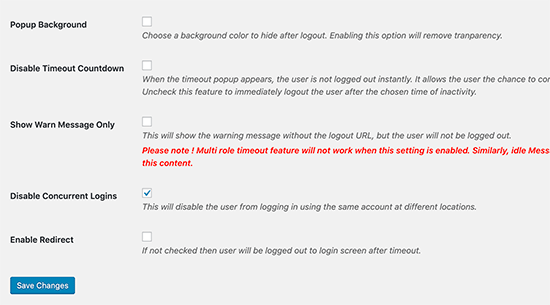The image depicts a user interface on a gray background with multiple options and settings presented in white checkboxes and textual prompts. The primary title reads "Pop-up Background" in bold black letters. Below are several settings with corresponding checkboxes:

1. "Disable Timeout Countdown" with an unchecked box to the right.
2. "Show Warn Message Only" next to another unchecked box.

Additionally, there's an important note in red text that states: 
"Please note! Multi-role timeout feature will not work when this setting is enabled. Similarity idle message cut off."

Following this, there are more settings:
3. "Disable Concurrent Logins," which is the only option checked with a blue check mark.
4. "Enable Redirect," accompanied by an unchecked white box.

At the bottom of these options, there is a prominent blue button labeled "Save Changes," allowing users to save any modifications made to these settings.